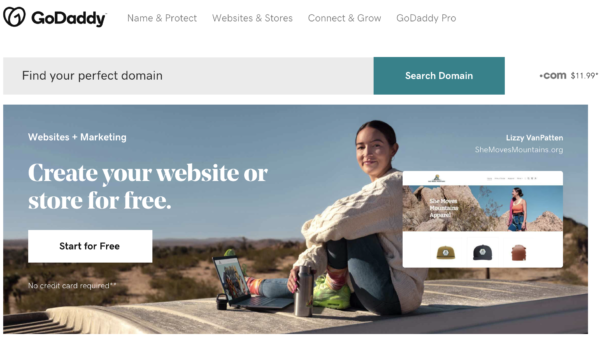This cropped screenshot captures the GoDaddy homepage in detail. At the top left corner, the "GoDaddy" name is displayed in black font, accompanied by the company's logo also in black. On the right side of the top navigation bar, four categories are listed in small grey letters: "Name & Protect," "Website & Stores," "Connect & Grow," and "GoDaddy Pro."

Below the navigation bar, a "Find Your Perfect Domain" search bar is prominently featured, with a blue "Search Domain" button to its right. On the far right, in small grey letters, ".com $11.99" is noted, accompanied by an asterisk.

Below this section is a large, vivid background photo showing a young woman sitting outdoors on top of a van, surrounded by nature. She has a laptop placed to her left side and is gazing directly at the camera. An overlay on the right side of the image displays a thumbnail of a webpage, likely representing her business hosted on GoDaddy. Above this thumbnail, in the top right corner of the photo, her name and website address are listed.

In the upper left corner of the photo overlay, "Website + Marketing" is displayed in small white letters. Directly below this text is a prominent white "Start for Free" button.